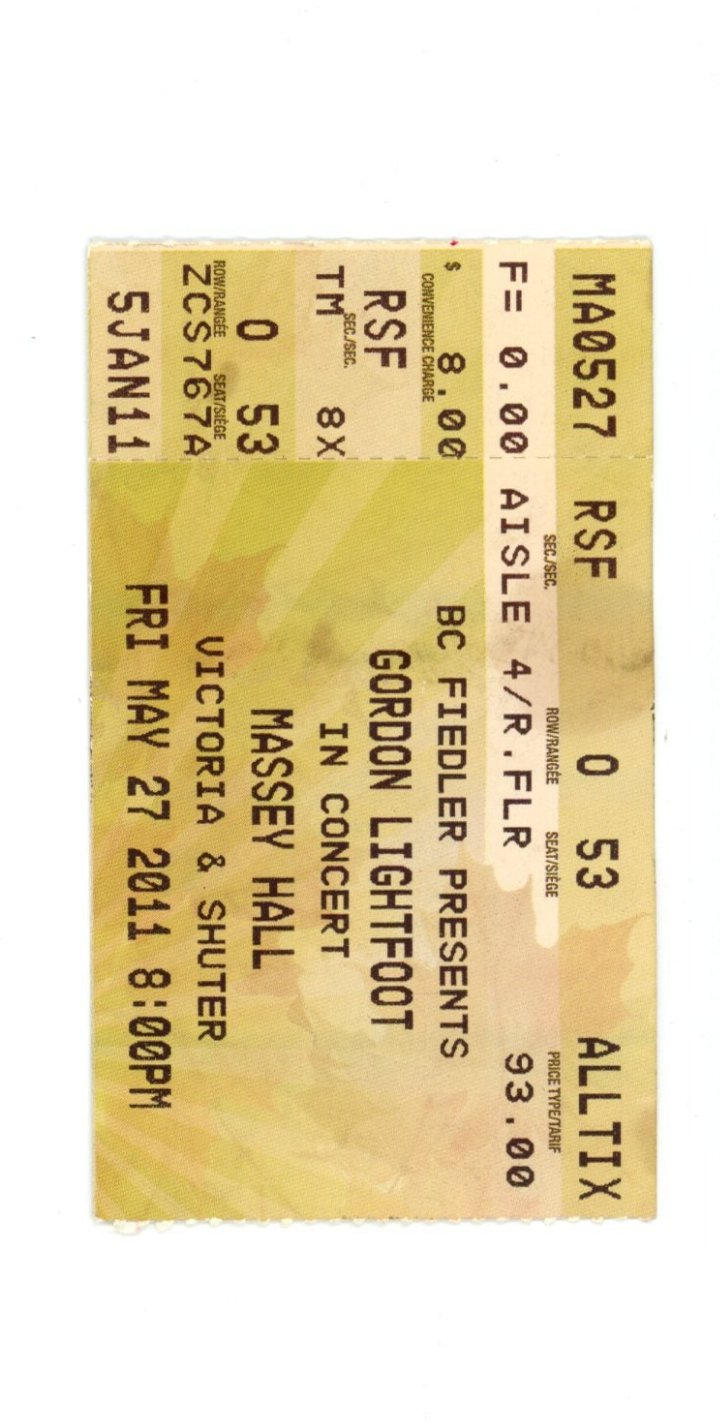The image depicts a used, yellow concert ticket with a faded background pattern for Gordon Lightfoot’s performance at Massey Hall, located at Victoria and Shudder. The concert took place on Friday, May 27th, 2011, at 8 p.m., and the ticket was priced at $93. The ticket was purchased from AllTickets, indicated by coding and tax figures on the upper left corner, specifically marked with "MA0527 RSF". The ticket, promoting "B.C. Fiedler Presents," shows the seat location as aisle 4/R on the floor. Part of the ticket has been torn off, likely by the gate attendant upon entry. The company Altix seems to have been involved with its distribution.